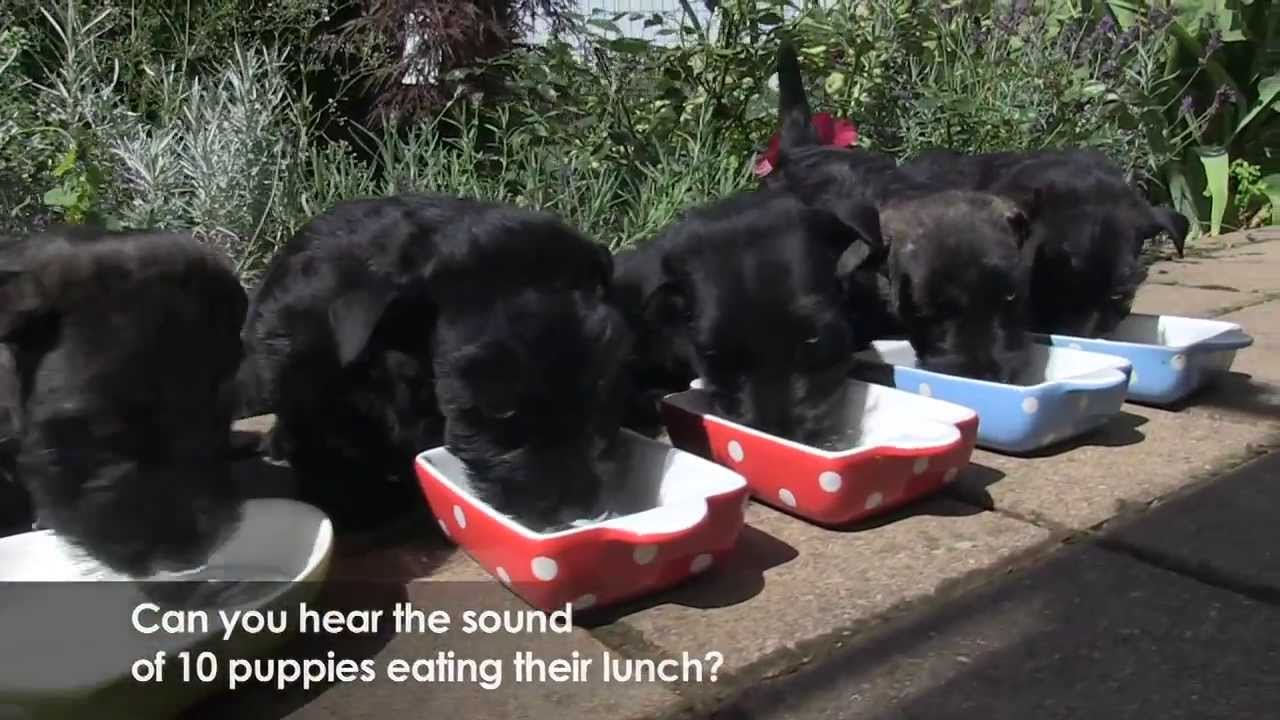The photograph, taken outdoors on a sunny day using natural lighting, captures a charming scene of five black puppies with soft fur and rounded, drooping ears eating from porcelain dishes. The image is horizontally rectangular, featuring a background filled with sunlit foliage, including various green leaves and possible tropical plants, with a hint of blue sky visible at the top. The puppies are positioned diagonally from the bottom left to the top right, each engrossed in their meal. They are arranged on a square-shaped stone patio or walkway with distinct, aligned stone tiles.

The puppies are feasting from square-shaped porcelain dishes, with two blue ones on the right, two red ones with white polka dots in the center, and a white dish on the far left. A semi-transparent black border with white text sits in the bottom left corner of the photograph, reading, "Can you hear the sound of ten puppies eating their lunch?". This whimsical caption adds a playful touch to the serene and picturesque setting.